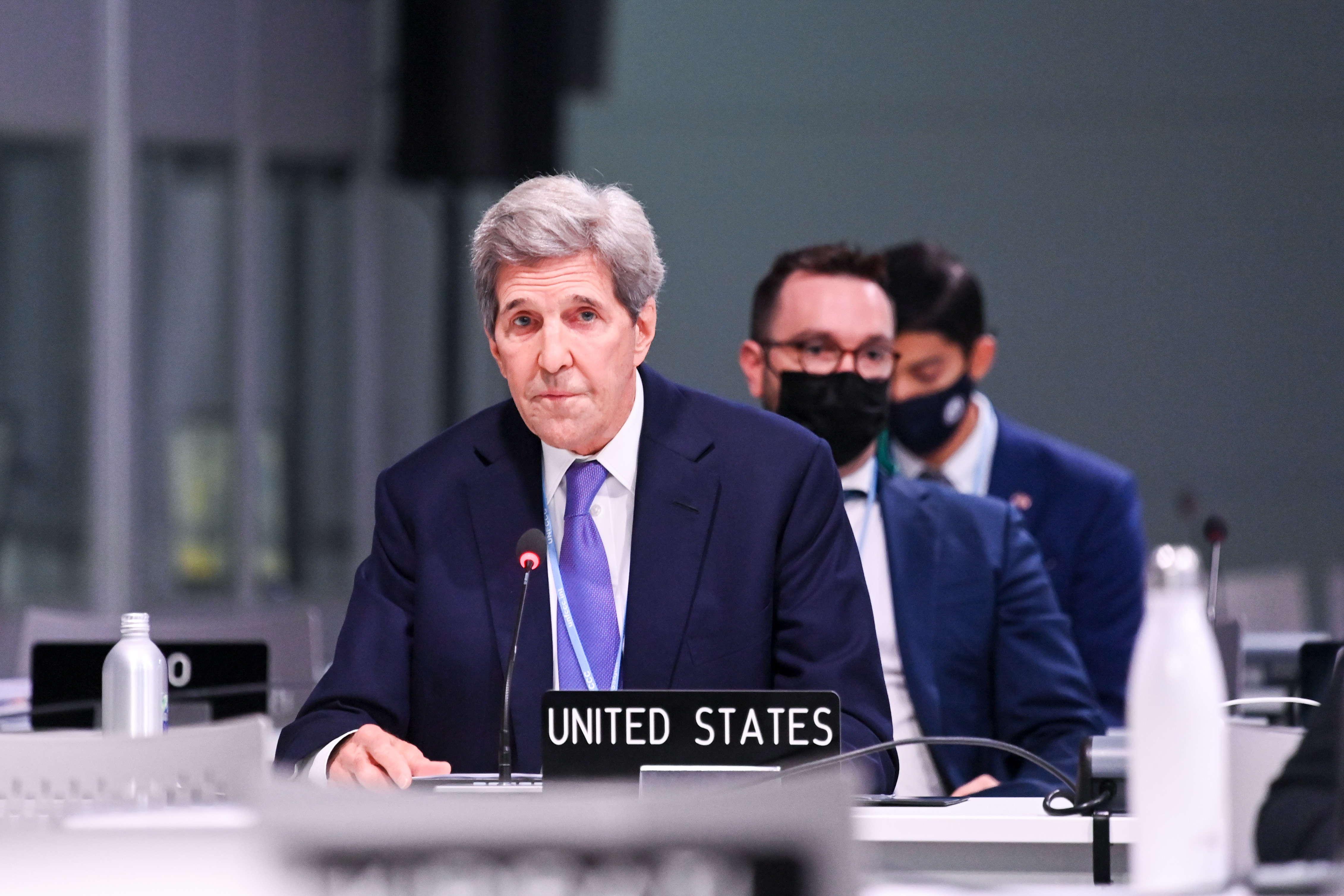This detailed photograph captures politician John Kerry, centered prominently, with a serious expression on his face. Kerry is dressed in a navy blue suit jacket and a slightly lighter blue tie. His gray hair contrasts with the dark, neutral tones surrounding him. In front of him is a microphone and a small black sign that reads "UNITED STATES" in bold white capital letters. On either side of this sign, there are white water bottles.

Behind John Kerry, two men are seated, both wearing navy blue suit jackets and black masks. The first man, positioned directly behind Kerry, has glasses and short dark brown hair, while the second man, who stands further back, has jet black hair. The background is composed of mostly neutral colors with various shades of blue. The setting appears to be a formal event, captured by someone with insider access. The men are seated at long white tables, adding a structured and official atmosphere to the scene.